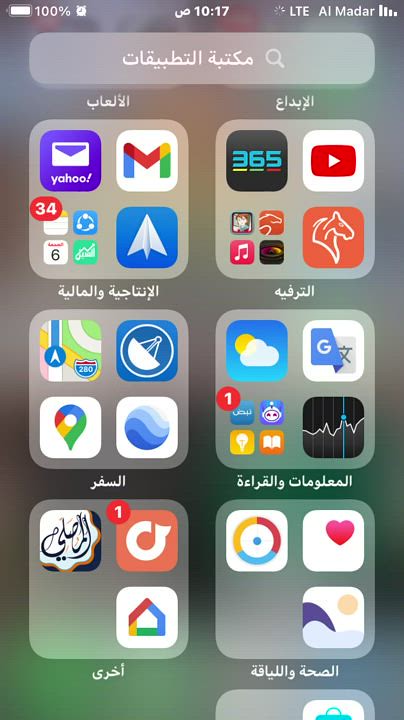The image showcases an iPhone home screen organized into seven distinct app groups, each labeled in Arabic. While the specific translation of these labels is not provided, it is clear that each group serves a particular function:

1. The first group appears to include communication apps, likely featuring a mail application.
2. The second group consists of entertainment apps, such as YouTube.
3. The third row from the top contains navigation applications like Maps and Waze.
4. Adjacent to the navigation apps, there is a collection of weather-related apps.
5. The bottom left group focuses on home automation, featuring apps likely related to controlling smart home devices.
6. Lastly, the bottom right group is dedicated to artistic apps.

The iPhone’s background is a blurred gradient, transitioning from green at the bottom to a more purple-hued top. Key status indicators are visible at the top of the screen, showing the battery percentage on the left, the current time in the middle, and the signal strength along with the carrier name on the right.